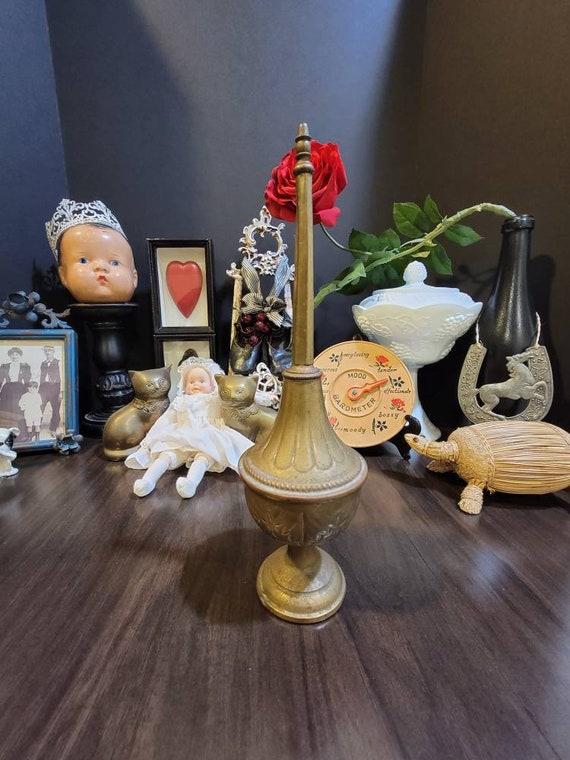The image features a dark brown, glossy, wood-like surface in the corner of a room, bordered by dark gray walls. Centrally placed is an antique golden-hued object resembling a carved wooden vase with intricate details, standing tall and tapering to a rounded point at the top. Adjacent and behind it are various objects: a black frame with a red heart, a black circular stand with a doll's head adorned with a crown, and a ceramic baby doll in a white dress and bonnet, flanked by two golden ceramic cats. To the left, a photo frame contains a black-and-white family picture from the 1800s, while to the right, a white ceramic dish with a lid sits next to an antique barometer. A striking dark gray bottle with a horseshoe and horse design etched on it stands prominently, with a stem featuring a red rose arcing above. In front of the bottle is a turtle crafted from wood or rattan, facing left. A clock-like plate with yellow detailing and red roses, and an array of green leaves further embellish the scene.